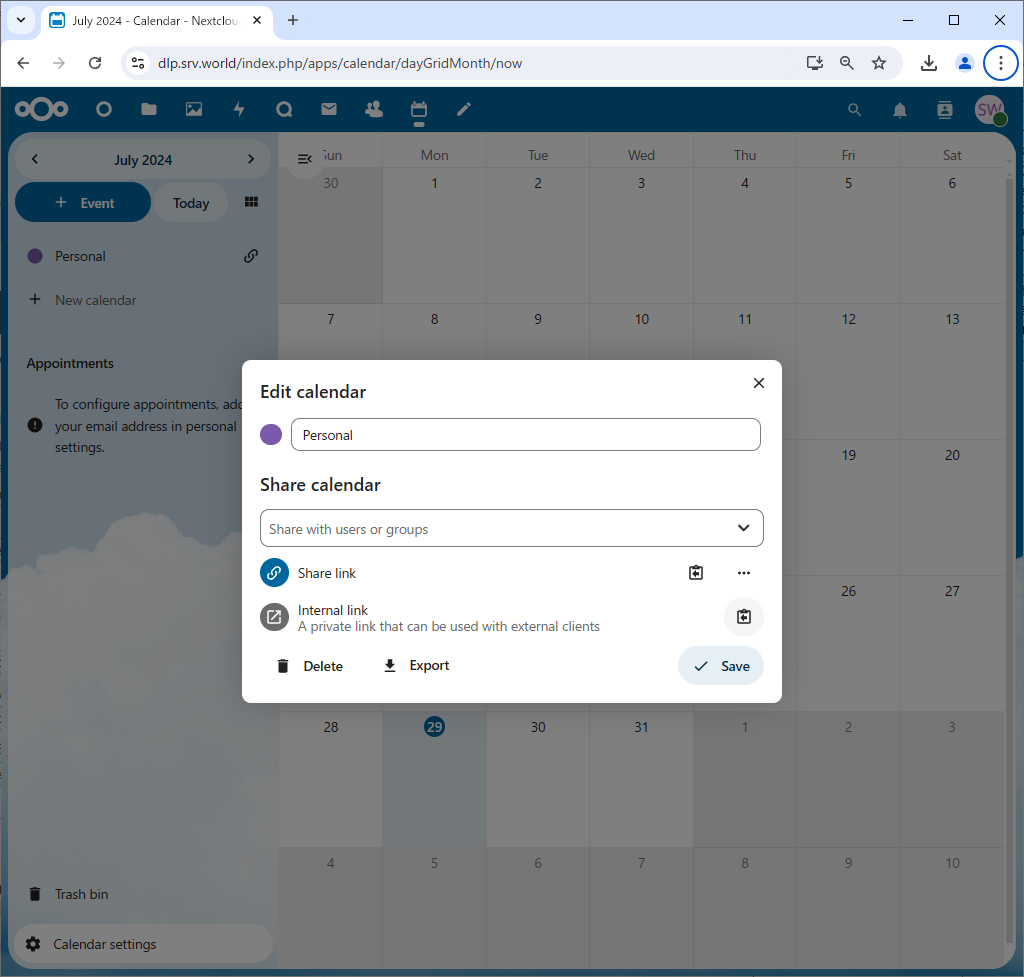In this detailed image, we see an open tab displaying a calendar from the web address "dlp.srv.world/nextcloud/index.php/apps/calendar/daygridmonth/now." The calendar appears to be from the month of July 2022, focusing specifically on the 27th. The days of the week are clearly labeled as Sunday, Monday, Tuesday, Wednesday, Thursday, and Friday. Prominent sections include options for "New Events," "Personnel," "Contact Birthdays," "New Calendar," "Appointments," and functionalities such as "Edit Name," "Edit Color," "Copy Private Link," "Export," and "Delete."

The visual design of the calendar incorporates various colors: blue for highlighted elements, yellow for important markers, black text for general content against a white background, and gray for additional accents.

At the top of the browser, the address bar features typical icons including the zoom-out magnifying glass, the share icon, the favorite (star) icon, as well as the controls for minimizing, maximizing, and closing the window. Notifications are also indicated, emphasizing the interactive and functional nature of this digital calendar interface.